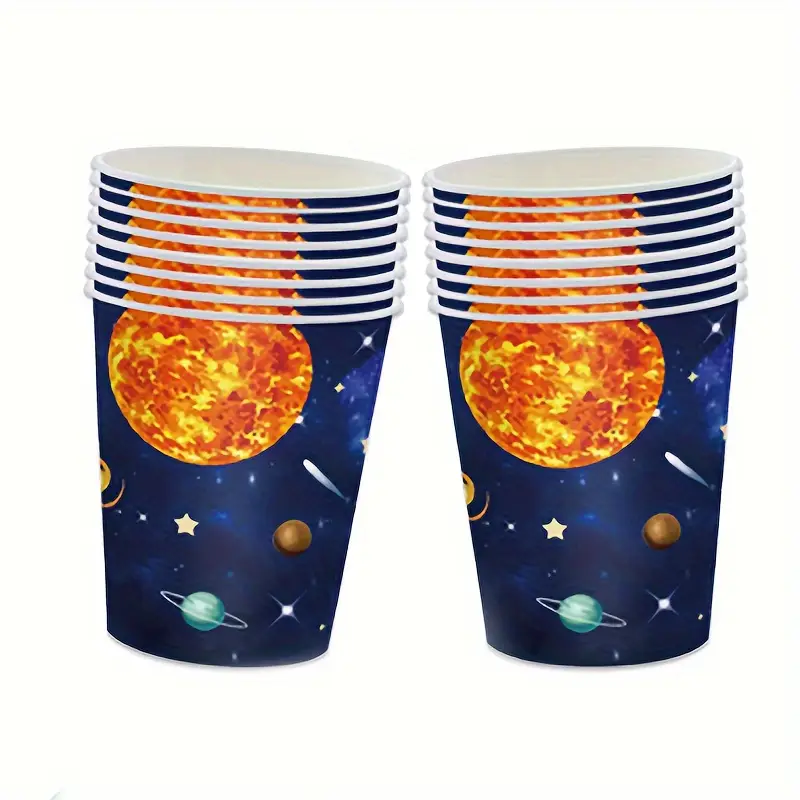The image features a stark white background showcasing two prominent stacks of paper cups. The exterior of these cups boasts a deep, midnight-blue hue reminiscent of a serene night sky. Adorning this celestial backdrop is an array of vividly detailed astronomical elements. A strikingly large moon, hued in vibrant shades of yellow and orange, dominates the design with its luminosity. Scattered across the cups are white stars varying in size and brightness, infusing the scene with a sense of depth and wonder. Among these stars are whimsical shooting stars and comets, each leaving delicate white trails in their wake. Adding to the cosmic tapestry are a series of planets: one is a rich, earthy brown, while another stands out with its blue body and distinctive white ring. A radiant star also catches the eye, its sharp points extending outward. The overall effect is a dynamic and captivating starry night, beautifully encapsulated on the surface of these paper cups arranged in two substantial stacks.